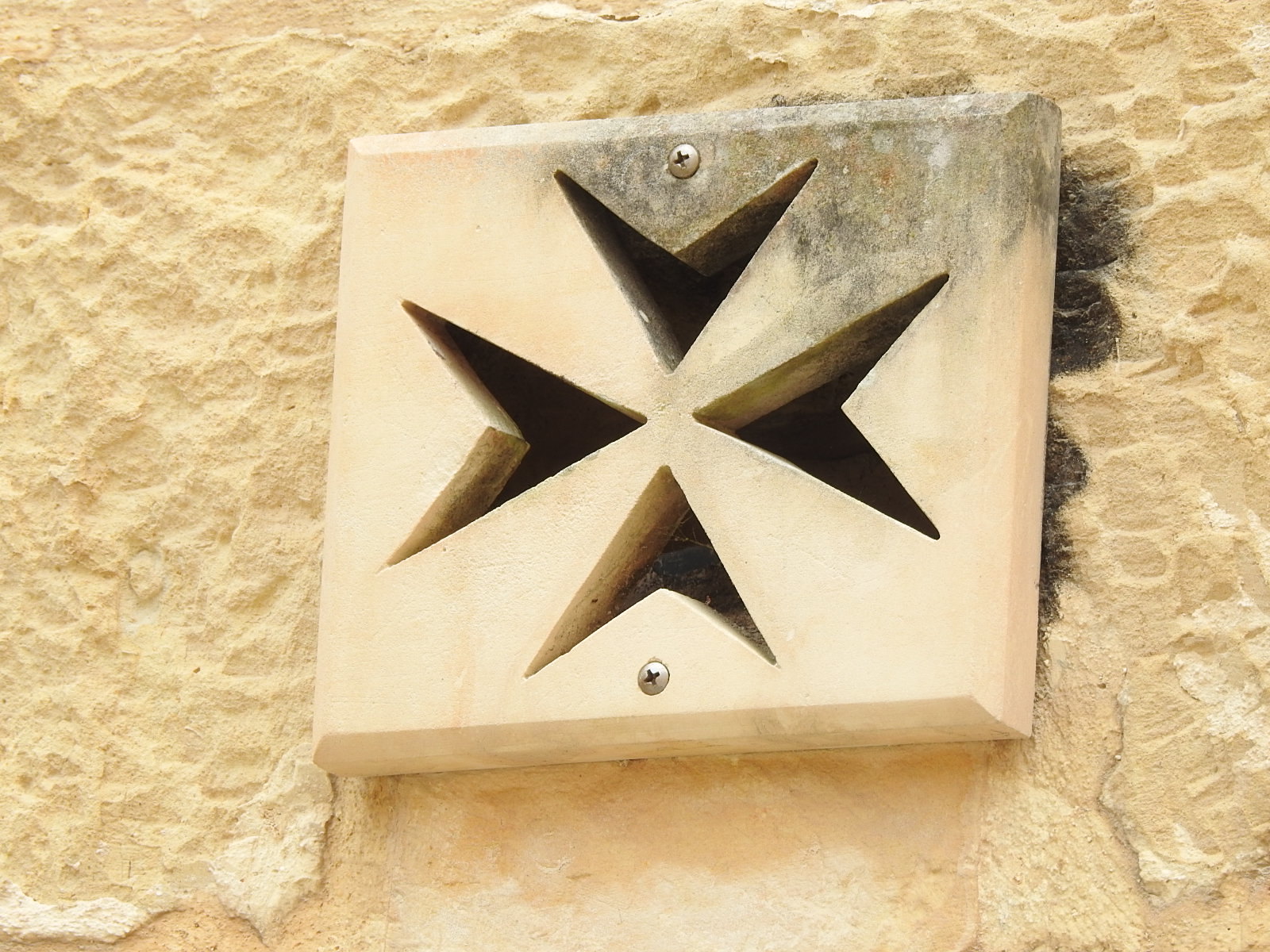The image depicts a detailed, mounted object fastened to a textured, yellowish-tan wall, likely made of sandstone or cement. The focal point is a yellow-hued wooden piece, featuring a distinct carved design resembling four arrowheads forming a cross-like shape. Each arrow points inward from the edges—top, bottom, left, and right—creating an angled, symmetrical pattern. The wooden piece is secured to the wall with two unpainted Phillips head screws, positioned opposing each other. The wall itself has a rough, raised texture, evoking a desert-like feel. Black smudges, possibly soot, are noticeable at the top right and beneath the wooden piece, suggesting the presence of smoke or a tunnel-like depth behind the carvings. The photograph, taken from a close range, draws attention to the tan and darker tan hues, complemented by the silver screws and the dark interiors of the arrow-shaped carvings. The ambiguous lighting leaves the setting—whether indoors or outdoors—undetermined.